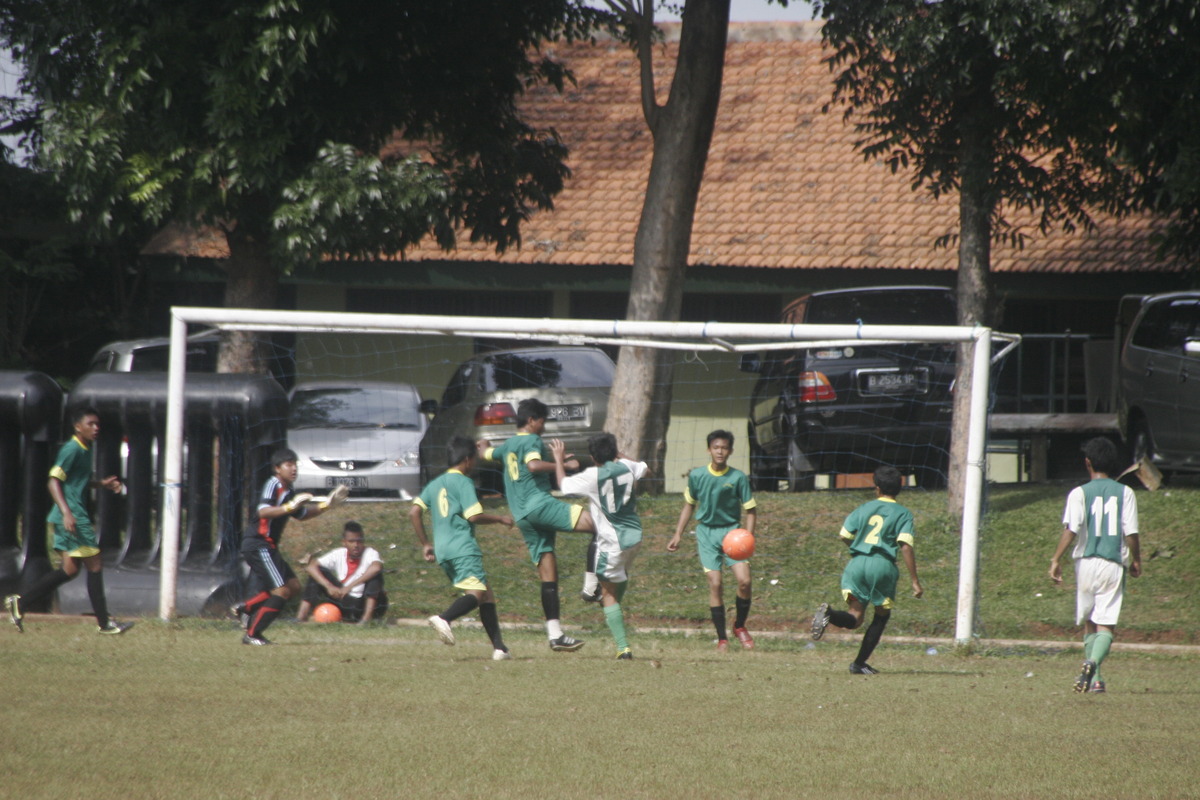This outdoor photo captures a lively scene of kids engaged in a soccer practice near the goalpost. There are nine to ten children, most of them with darker skin tones, dressed predominantly in green sports outfits with yellow numbers, and a few in mixed white and green jerseys. An orange soccer ball stands out against the green field. One child is sitting on the ground, possibly on the sideline, with the ball in front of him, while the rest are dynamically chasing or contesting for the ball. The goalie, poised to kick off, reacts energetically to the game. In the background, there's a row of parked cars reminiscent of a parking lot and a two-story building with orange brickwork, likely a school. Several trees with lush green leaves frame the area, adding a touch of nature to this energetic sporting event.